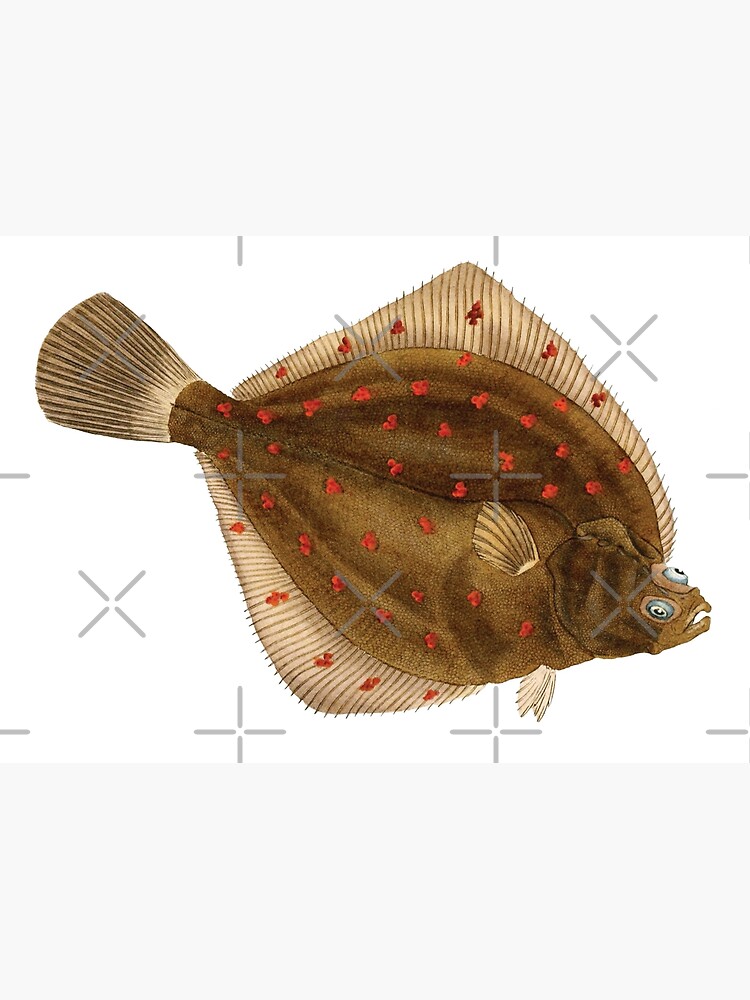This is a detailed illustration, likely watercolour, of a peculiar, flat-bodied fish with a unique design. The body of this fish is quite flat, reminiscent of a stingray, and has an overall oval shape. Its colouration is primarily brown, adorned with numerous yellow and red dots across its body and fins, which contribute to its distinctive appearance. The fish features two massive, spade-shaped fins, unusually positioned right behind its head, extending across the top and bottom of its body. It's also equipped with a sizable tail fin. The fish's eyes are oddly placed on its head, facing upwards, giving it a rather bizarre facial expression. The image appears to be watermarked with computer-generated gray crosses and X's over a white background, perhaps indicating it is intended for a scientific publication or journal. Additionally, there are two gray rectangles situated at the top and bottom of the image, enhancing its peculiar, almost scientific presentation. The combination of these features suggests the fish might be a deep-sea species, purposefully illustrated to emphasize its strange morphology.